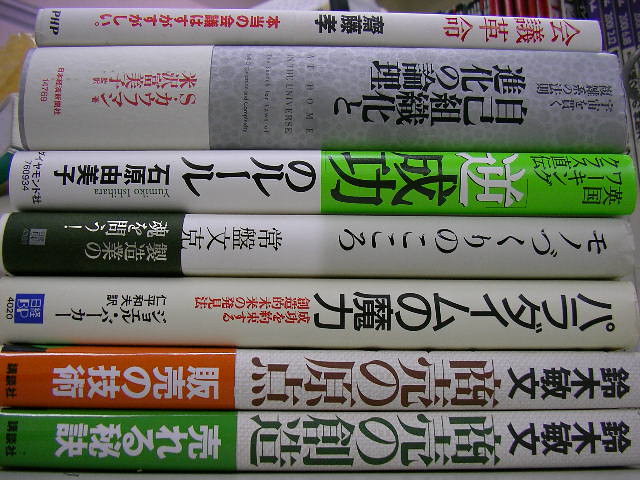This image features an extremely close-up shot of a stack of seven hardcover books, arranged horizontally with the spines facing outwards. The books are stacked from top to bottom, not left to right, making the spines the focal point. The text on the spines is in Japanese, utilizing mostly black characters but also featuring red, green, and orange lettering. 

From top to bottom, the first book has a white spine with a neon green top section and Japanese text in black and dark green. The second book features a white spine with an orange top section, bearing black, red, and white text. The third book is entirely white with a mix of black and smaller red text, along with a small dark blue square containing Japanese characters and the numbers "4020" in black. 

The fourth book starts with a light gray section, transitions to white with black text in both sections, followed by a dark green area with golden characters, and a small light gray square containing light gray numbers. The fifth book’s spine is primarily light green, featuring black, white, and more black Japanese text, followed by a white section with a larger set of black characters and the numbers "760934" at the edge. 

The sixth book begins with light gray spanning more than half its spine, which then transitions to white with red and black text, with the numbers "14769" at the end. The seventh and final book's spine is white, featuring red text at both the top and bottom with black text in between, ending with black text spelling out "PHP". 

The relative thickness of the books varies; the sixth book is the thickest at about three times the thickness of the others, while the top book is slightly thinner than the rest, except for the widest. The image is so close that it emphasizes the details in the colors, text, and textures on the spines, showcasing the vibrant and varied design elements of the books.